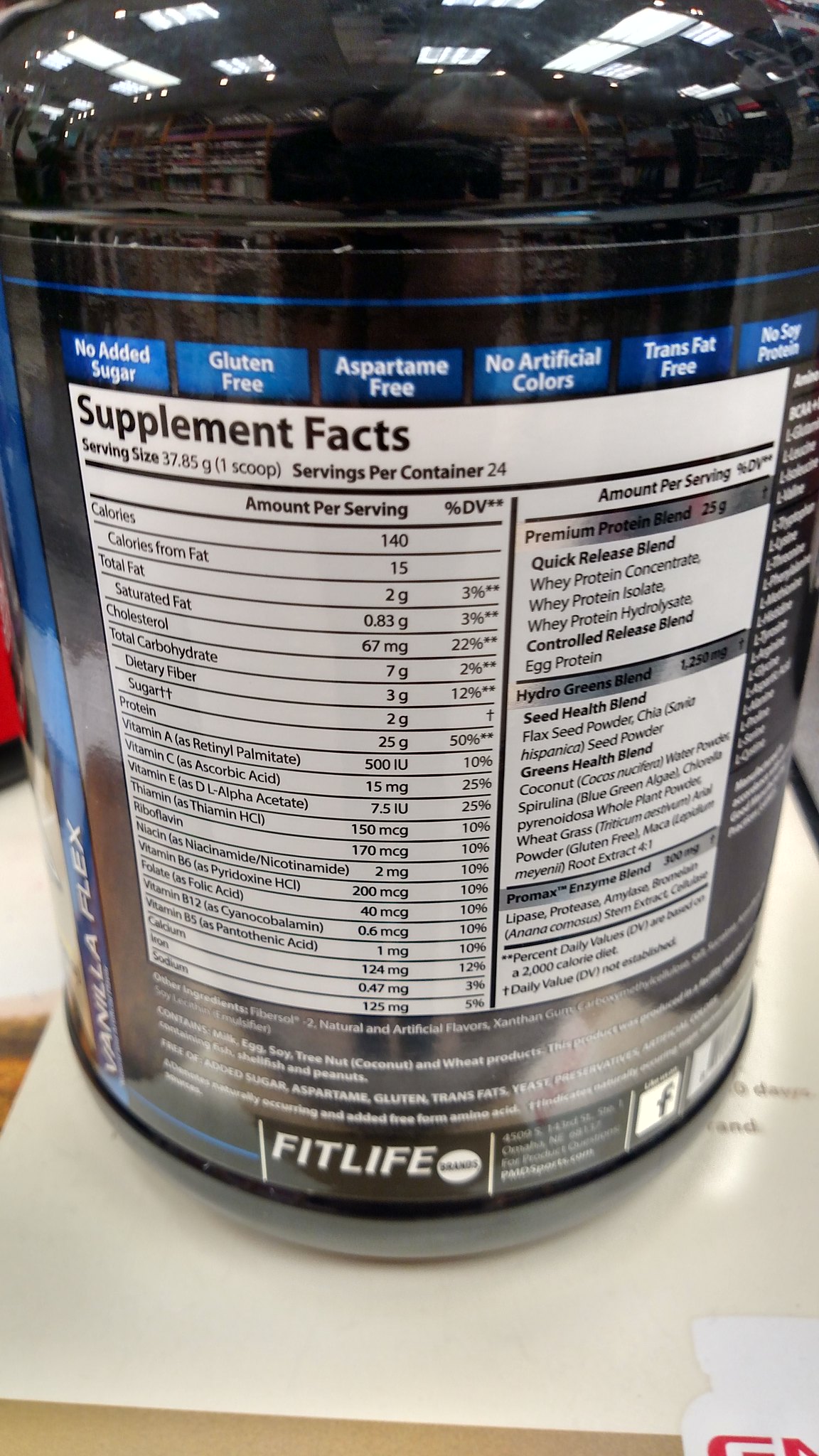This image depicts the back of a FitLife product container, resembling a can made from semi-translucent, smoke-white plastic that peeks out below a dark-colored label with blue elements. The label prominently features a blue line with the product name "Vanilla Flex." The container has a rounded, screw-on lid that is highly reflective, indicating store lighting, likely halogen, with visible shelves and ceiling panels in the background. 

On the label, multiple blue informational boxes state: "No Sugar Added," "Gluten-Free," "Aspartame Free," "No Artificial Colors," "Trans Fat Free," and "No Soy Protein." A large white box on the back provides detailed supplemental facts: serving size is 37.85 grams (one scoop), with 24 servings per container. Nutritional details include 140 calories (15 from fat), 2 grams of total fat (3% DV), 0.83 grams of saturated fat (3% DV), 67 milligrams of cholesterol (22% DV), 7 grams of total carbohydrates (2% DV), and 3 grams of dietary fiber (12% DV). At the bottom, "Fit Life" is clearly written in white letters. The container is placed on a piece of paper, with the top corner of a GNC label partially visible, indicating the vitamin company.